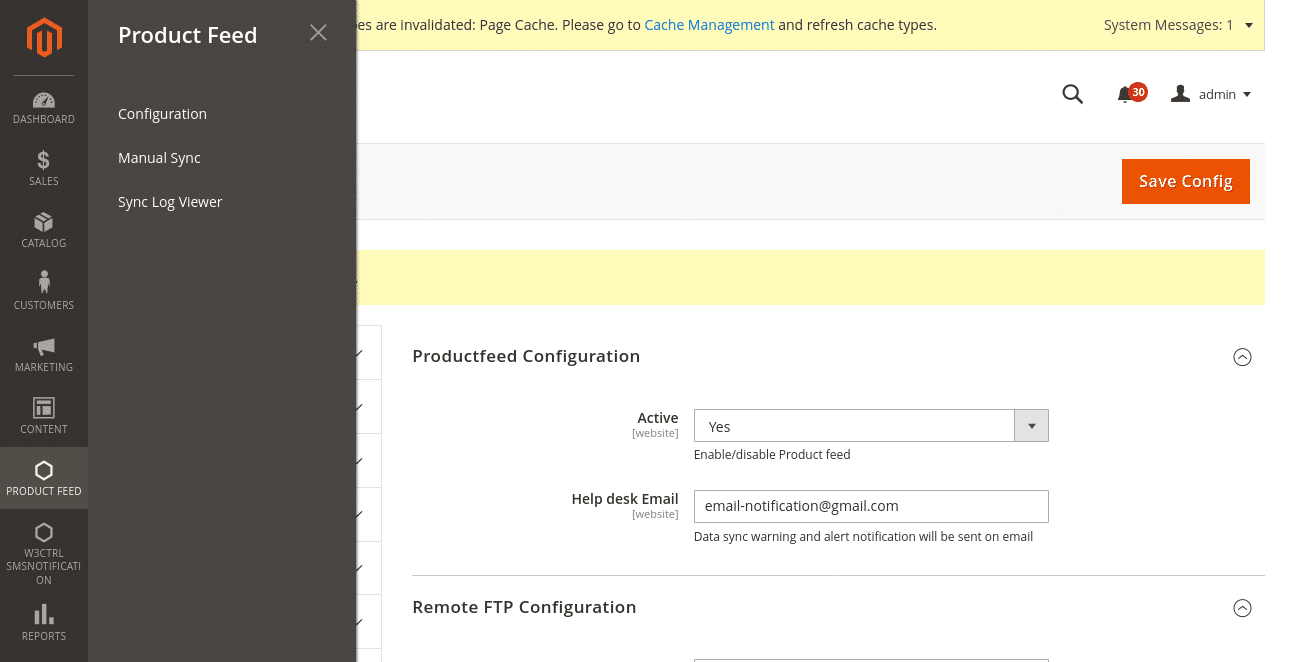The image displays a detailed screenshot from a website's user interface, prominently featuring a pop-up window overlaying the main page content. 

On the left side, there is a vertical navigation menu with a darker background color. At the top of this menu, an orange logo is visible. Below the logo, the menu items are listed in the following order:

1. Dashboard
2. Sales
3. Catalog
4. Customers
5. Marketing
6. Content
7. Product Feed (highlighted)
8. W3CTRL
9. SMS Notification
10. Reports

The pop-up itself has a grayish-brownish background. At the top of the pop-up window, there is an orange logo. The menu items within the pop-up are listed as follows:

1. Product Feed (highlighted)
2. Configuration
3. Manual Sync
4. Sync Log Viewer

In the upper right-hand corner of the pop-up, there is an "X" for closing the window.

The background page behind the pop-up has a white background with yellow banners located at the top and middle sections. The yellow banner at the top features text, part of which reads: "Art Invalidated, Page Cache. Please go to Cache Management and refresh cache types." 

On the right side of the page, there is a section titled "Existing Messages," followed by a magnifying glass icon, "30 new messages," and an "Admin" dropdown menu. Additionally, there is an orange square button with white text reading, "Save Config."

Underneath the "Save Config" button is another section with the label "Product Feed Configuration." This section includes the following details:

- "Active: Yes"
- "Help Desk Email"
- An email address (obscured in this description).

In summary, the screenshot captures the detailed layout and overlapping elements of a website's administrative interface, including the navigation menu, a central pop-up window with various configuration options, and sections of the main page with notification messages.